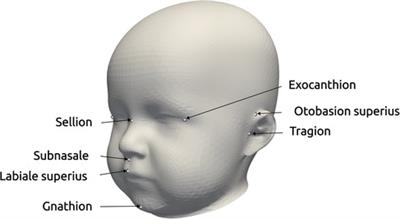The image presents a detailed 3D model of a baby's head with a white background, meticulously labeled with various anatomical terms. The head is bald, spherical in shape, and rendered in shades of gray, giving it a computer-generated appearance. Black labels identify key parts of the face and head. 

On the left side of the head, labels include "Salien" near the eye area, "Subnasal" and "Labiale Superius" below the nose, and "Nasion" around the chin area. On the right side, the terms "Exocanthion" (edge of the eye), "Autobasion Superius" (above the ear), and "Tragion" (center of the front of the ear) are noted. Additionally, "Cilion" marks the top of the nose, "Subnasal" is again indicated below the nose, and "Labiale Superius" signifies the top center of the lip, while "Gnathion" denotes the chin.

The eyes are depicted as white indentations, while the mouth, nose, and ears are distinctly labeled but abstractly rendered, adding to the surreal, almost ethereal quality of the model. This detailed labeling aids in the study and identification of facial anatomy, presented in a clear and concise manner against the stark white background.